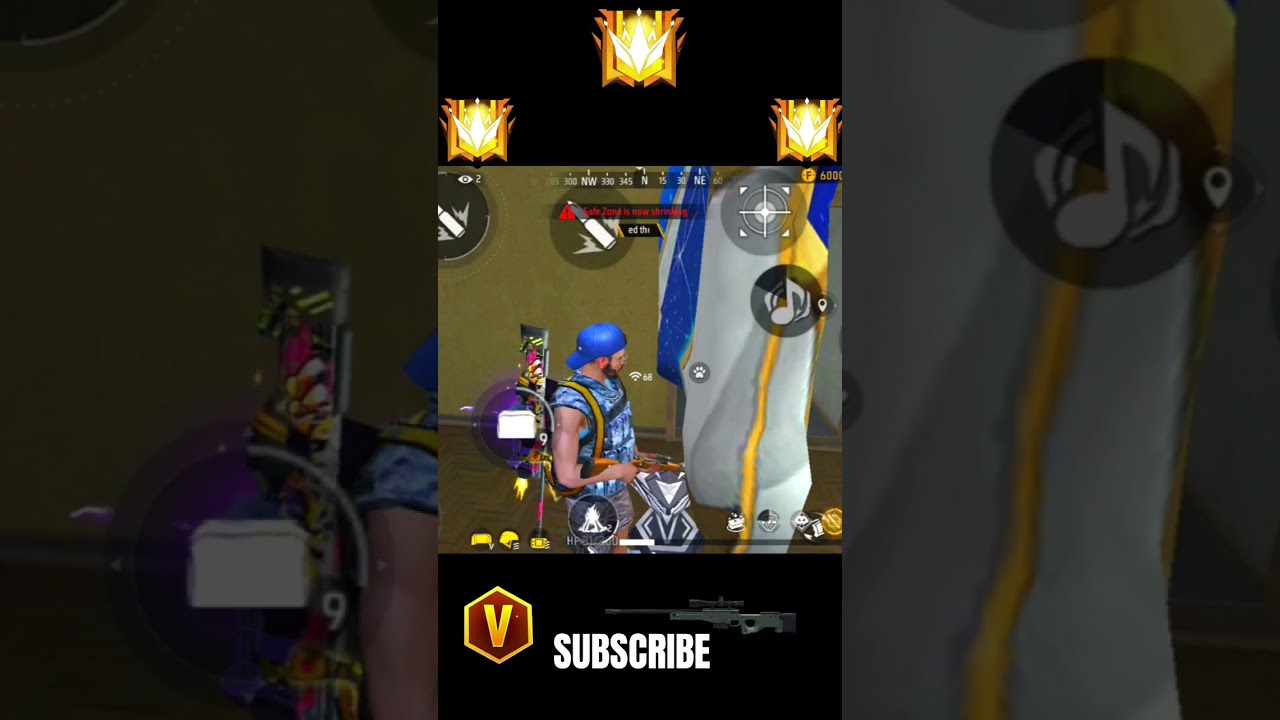The image appears to be a screenshot from a video game taken on a mobile device. It prominently features a Caucasian man in the center, who appears to be a hunter or military figure. He is wearing a blue camouflage shirt with cut-off sleeves, a backwards blue baseball cap, gray and white camo pants, and he has a thick brown beard and mustache. The man is walking on a carpeted area and is holding a light brown wooden sniper rifle with another gun, possibly a fancy purple and white painted one, strapped to his back.

Surrounding the man in the screenshot are various game UI elements. At the top of the image are three gold crown symbols. To the right of the man, there appears to be a mysterious white object, possibly a T-shirt or target. Below the man, some icons are visible, including a hexagonal badge with a golden trim, a burgundy interior, and a golden 'V' in the center, and another icon showing a sniper rifle. To the left of the man is a file folder icon with the number nine next to it, possibly indicating ammunition or inventory. 

The entire image has a black border, with the word "subscribe" prominently displayed at the bottom along with the image of a gun and the letter ‘V’. The background features a mix of colors including black, yellow, orange, white, blue, light blue, purple, and gray, suggesting an action-packed scene in a visually dynamic game.